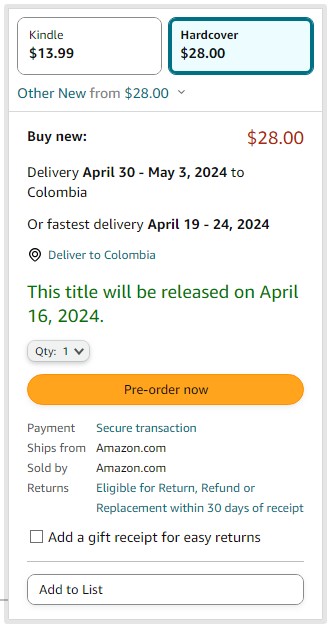This screenshot is taken from the Amazon US website, as indicated by the prices displayed in dollars. The screenshot does not show the title or image of the book, but the available purchasing options and pricing details suggest that it is possibly a book. The Kindle version costs $13.99, and the hardcover edition is priced at $28. There are also new copies available starting at $28.

The book is set for release on April 16, 2024, and can currently only be pre-ordered. The anticipated delivery dates are between April 30 and May 3, 2024. The buyer's location appears to be in Colombia, as the estimated delivery time is specific to there. The transaction is secured, and the book will be shipped directly from Amazon.com, indicating it is from the global branch.